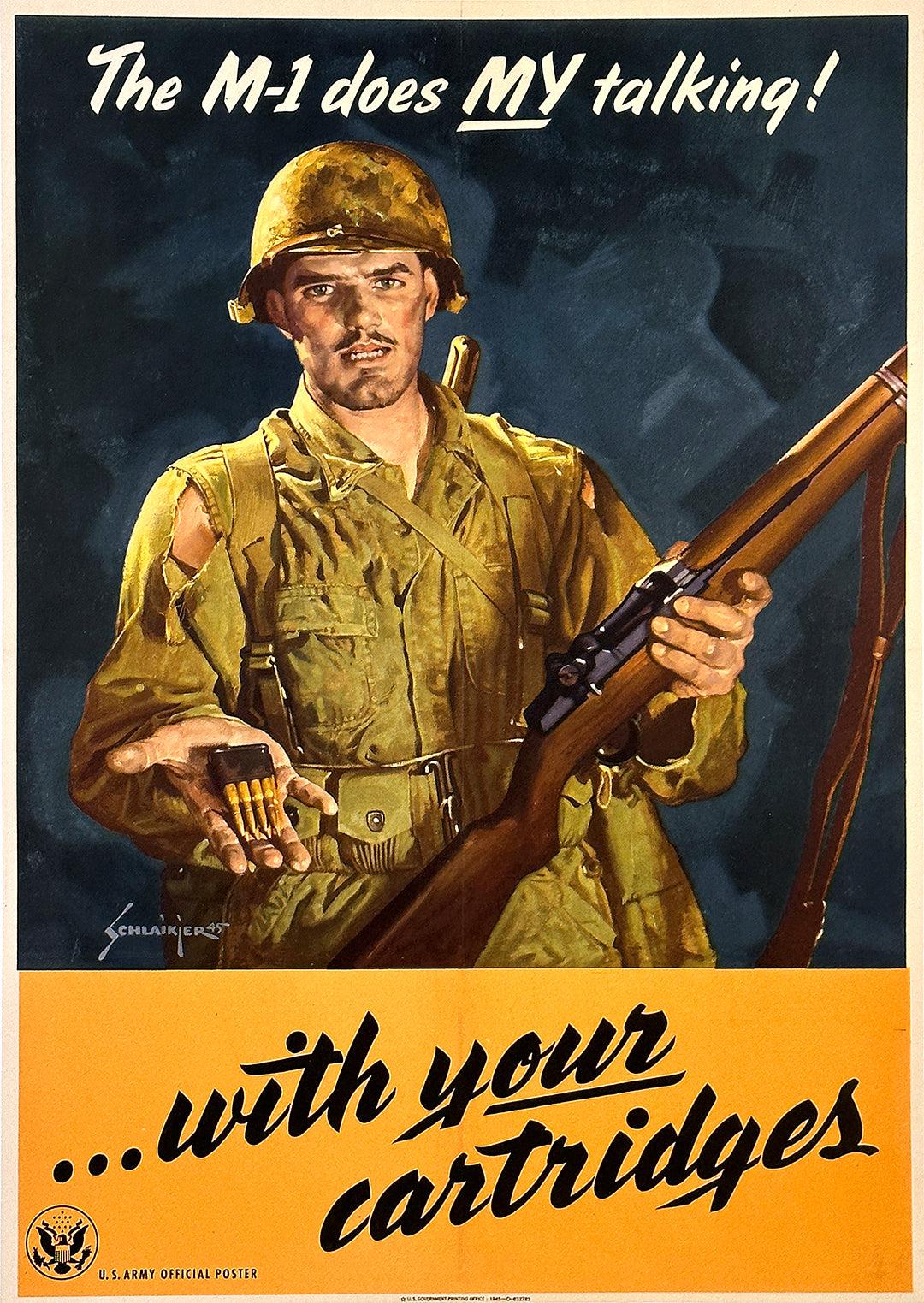This U.S. Army official World War II propaganda poster prominently features a detailed painting of a soldier in olive green fatigues and a helmet. The soldier, who appears to be in his mid-20s with a thin black mustache and a slightly stubbly beard, is holding a brown rifle with a leather strap dangling from it in his left hand, while his right hand, palm side up, displays four bullets. His uniform is notably torn on each shoulder, adding to the gritty appearance. The top two-thirds of the poster, set against a dark blue-gray background, showcases the bold white text, "The M1 does my talking!" with "my" underlined and capitalized for emphasis. Below the soldier, a yellow section features the text, "...with your cartridges," with "your" underlined. In the bottom left corner, there is a small dark emblem resembling the presidential seal, with the text "U.S. Army official poster" accompanying it.